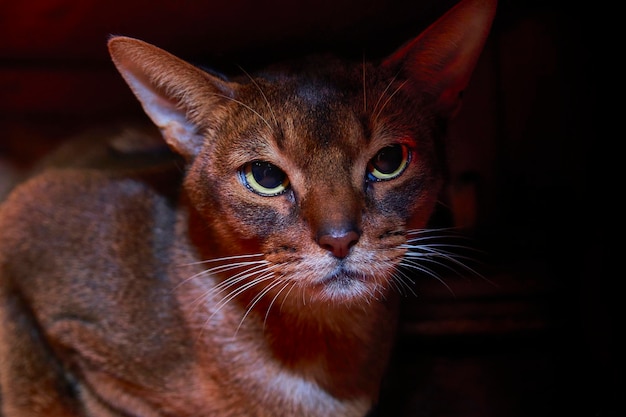This is a detailed photograph of a beautiful cat, situated in a very dark background that accentuates its features. The cat has a dark brown coat with a patch of lighter brown and white fur around its mouth, showcasing its mature and poised demeanor. Its nose is a striking red, dusted with dark fur around it, and long, white whiskers flare out to the sides and top of its head. The cat's large ears are diagonally pointed up, with hints of reddish coloring and a tiny glimpse of pink inside. 

The most captivating aspect of the cat is its eyes. The pupils are significantly dilated, making them appear almost entirely black, with a subtle green hue around the edges, conveying a sense of life and mystery. Despite its somewhat skeptical and slightly concerned expression, the cat's eyes also reflect a certain calmness, possibly sensing or awaiting something. 

The lighting suggests it's in total darkness, providing a dramatic contrast to its dark fur, and highlighting its muscular shoulder that is crouched on the ground, ready to pounce, giving it an aura of readiness and alertness. This blend of features makes it challenging to determine if it's a domestic breed or a wild feline, adding to the mystique of this serene and enigmatic creature.